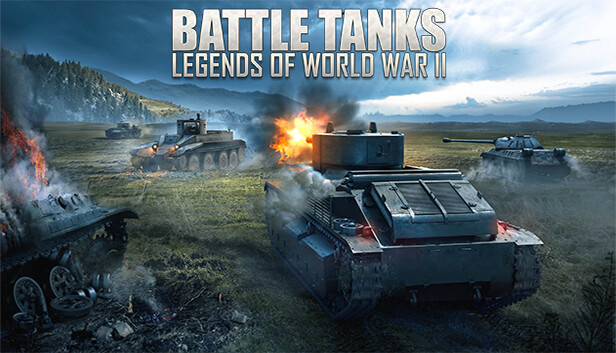The image appears to be a vibrant screenshot from a video game titled "Battle Tanks: Legends of World War II," prominently displayed in silver, all-capital letters at the top center. The scene captures an intense tank battle set on a broad, grassy battlefield framed by distant hills and a dark, cloudy sky. Dominating the foreground slightly right of center is a large, silver tank with thick treads, actively firing its turret, with flames erupting from the gun barrel. Surrounding this central tank are several others: to its right, a smaller tank trails smoke, and in front, two additional tanks are visible further back. On the far left lies a charred, burning vehicle with its wheels dislodged, adding to the chaos of the scene. The detailed and dramatic tableau evokes a sense of historical warfare amidst a visually dynamic and foreboding landscape.